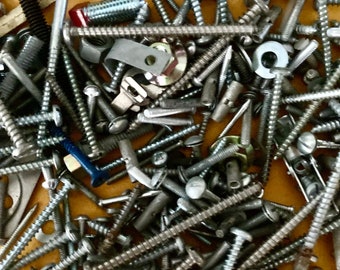The image is a detailed close-up of a jumbled collection of various fasteners, including primarily screws but also nails, washers, tacks, and metal picture-hanging hardware. The background is an orangey-yellow surface, which contrasts with the mostly silver-toned metal objects, although you can spot a few dark blue nails and pewter-colored washers. The screws come in different shapes and sizes—some are flat-headed, others star-headed, and there are also rivets, bolts, and wing nuts visible among them. Notably, there are a few black screws scattered, particularly in the top left corner and the middle of the image. The screws vary in length, with some as long as six to eight inches and others as short as three inches. While many of the screws are new and shiny, some appear worn and rusty. The image is sharply detailed, capturing every minute aspect of the fasteners against the vibrant yellow backdrop.